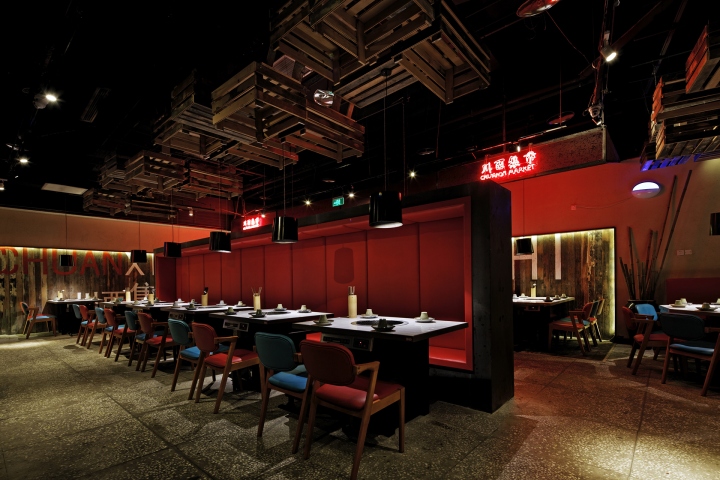The photograph presents the interior of a dimly lit, Asian-themed barbeque restaurant adorned with distinct neon signage in both Chinese and the Latin alphabet. A central vertical divider, embellished with wooden crate-like ornamentation, runs through the seating area. On one side of this divider, continuous red leather couches offer communal dining, while individual blue and red chairs line the other side. Circular barbeque grills are embedded in the white tabletops, enhancing the communal dining experience. The tables are situated close together, emphasizing an intimate dining setup. A consistent red hue pervades the scene, evident in the ambient lighting, seating, and divider, creating a warm and inviting atmosphere. The restaurant appears void of customers or staff, offering an unobstructed view of its architectural elements and grayish-green concrete tiled flooring.